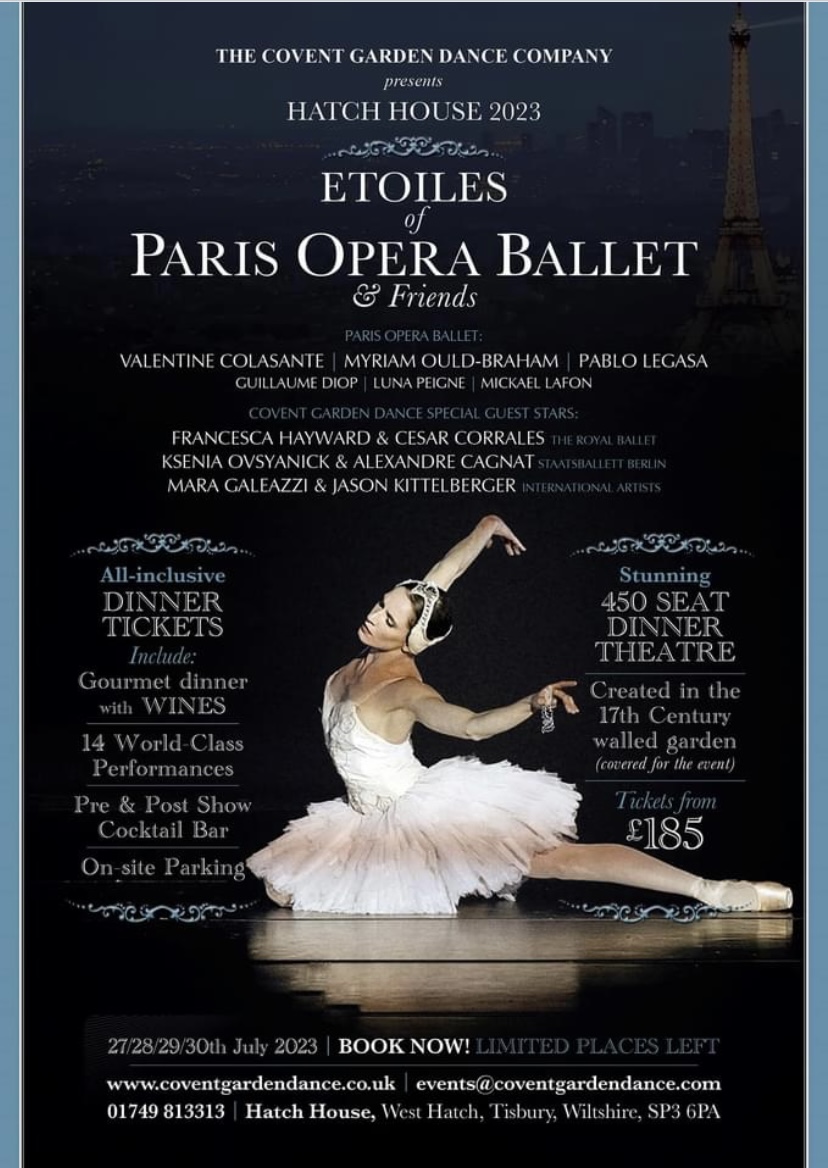This poster advertises a captivating ballet performance at Hatch House in July 2023. The black background highlights the elegant white text announcing "The Covent Garden Dance Company presents Hatch House 2023, etoiles of Paris Opera Ballet and Friends." At the center, a graceful ballerina poses with one leg outstretched and arms curved gracefully, clad in a delicate light pink tutu with a toile skirt and toe shoes. Her hair is styled in a bun adorned with a small white crown, and her eyes appear to be closed in a serene expression. The top of the poster subtly features Parisian skyline elements, including a shadowed Eiffel Tower, all in a dark blue tint.

Details on the left specify the luxury of the "All-inclusive dinner tickets," which provide a gourmet dinner with wines, access to 14 world-class performances, and pre- and post-show cocktail bars, along with on-site parking. To her right, it describes the "stunning 450-seat dinner theater centered in a 17th-century walled garden," with tickets starting at £185. The dates 27th, 28th, 29th, and 30th of July, 2023, along with a call to "Book now," are prominently displayed at the bottom. Additional fine print gives event and location specifics, ensuring all pertinent details are elegantly encapsulated in this visually striking advertisement.